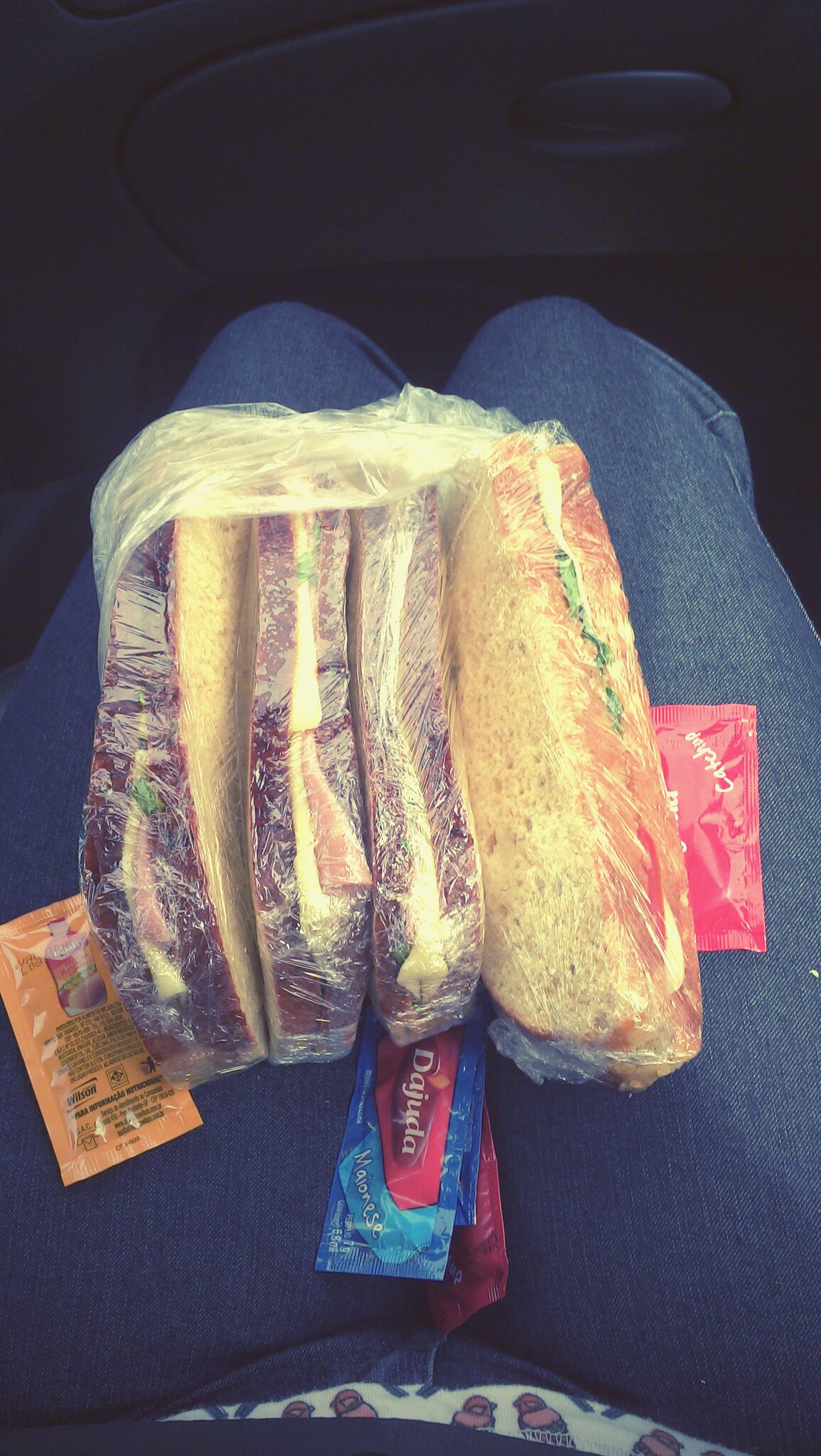This detailed color photograph captures the top-down view of a person sitting in what appears to be a car, evident from the visible seatbelt across their waist and a dark glove compartment at the top of the image. The person's legs, clad in blue jeans, stretch out up to the knee, with a small portion of their white, patterned blouse peeking out at the bottom. The pattern on the blouse sports orange birds.

Resting on the person’s lap are four cellophane-wrapped sandwiches neatly arranged in a row. The three sandwiches on the left feature dark brown crusts and contain a mix of cheese and deli meats, likely roast beef or turkey. These three similarly shaped sandwiches reveal little more than their crusts and fillings peeking through the clear wrapping. The fourth sandwich on the right stands out with a lighter, broader crust and appears to include components like lettuce and possibly tomato, along with meat and cheese.

Scattered around the sandwiches are an assortment of condiment packets in various colors. To the left of the arrangement is an orange packet, speculated to be some type of hot sauce. Between the person's legs and beneath the sandwiches are a blue packet with a red banner, possibly labeled "Deason Dog AJ UDA," and a couple more packets in blue, orange, and red shades. The background of the image remains dark, highlighting the casual snacking setup on the lap of the seated individual.